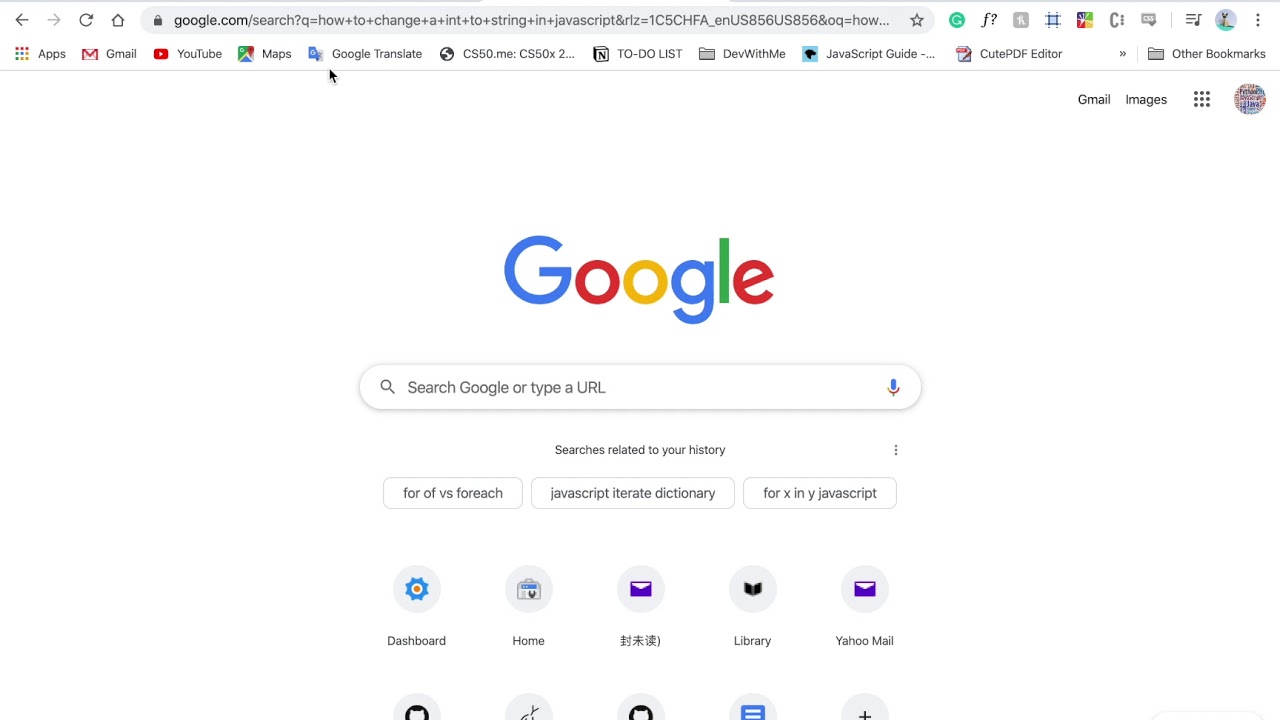The image depicts a Google search page as seen on a web browser. The central focus is the iconic Google logo, displayed prominently in its traditional blue, red, yellow, and green colors. Situated at the top of the page is a white header featuring various tools and options, such as Apps, Gmail, YouTube, Maps, Google Translate, and a to-do list. On the far left of the header, a shaded gray area shows "Google.com."

Below the header is the familiar Google search bar, inviting users to "Google search or type a URL." A microphone icon is located on the right side of the search bar, indicating voice search functionality. Directly beneath the search bar, a note mentions that the results are related to the user's search history.

Further down, four distinct search suggestions appear in white boxes, including comparisons like "four of vs. for each in JavaScript," and other related terms like "literate dictionary" and "for X in JavaScript."

Accompanying these search results, a series of images are displayed. These images include a dashboard, a home icon, an email or message symbol in a different language, a library, and a Yahoo Mail icon, along with several other partially visible images. The page is rich with various icons and symbols situated above the header, adding to its informational and navigational elements.